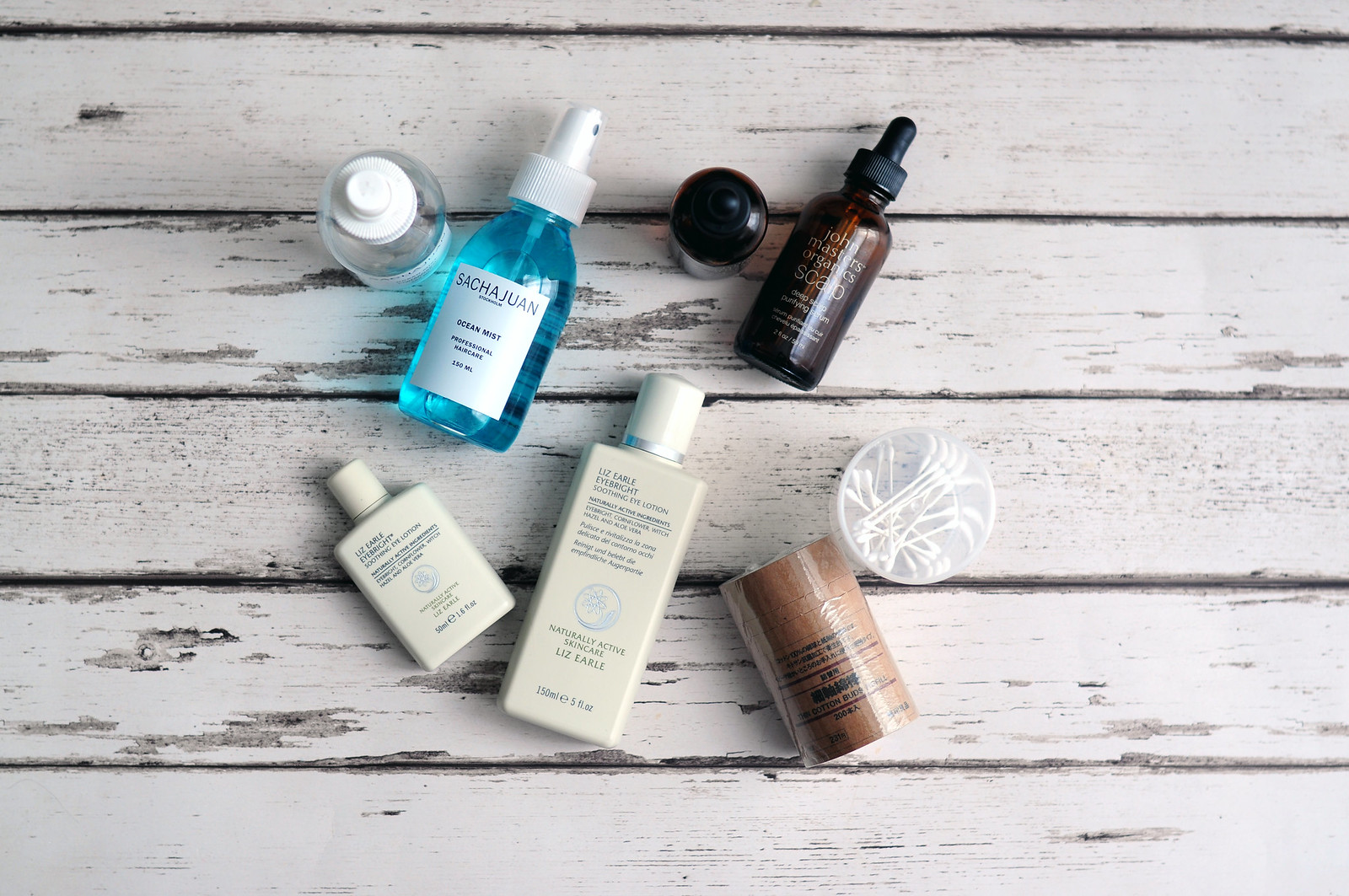The image captures a variety of toiletry items arranged on a distressed wooden surface, possibly a table or countertop, composed of white-painted slats showing signs of wear. Among the items is a clear spray bottle filled with blue liquid, labeled "Satchewan," though the smaller print is unreadable. Two white, rectangular bottles lie on their sides, featuring capped tops—again, the labels are too faint to discern. A cylindrical brown plastic container, possibly deodorant, is also present. Nearby, a round clear container holds cotton tip applicators, recognizable under the brand name "Q-tips." Additionally, a round bottle with a dropper lies on its side next to a dark-colored, dropper-topped bottle standing upright. Another clear round bottle, topped with a white cap, stands to the side, resembling a spray bottle. The assortment of items evokes a rustic yet organized feel, capturing the essence of everyday personal care essentials.